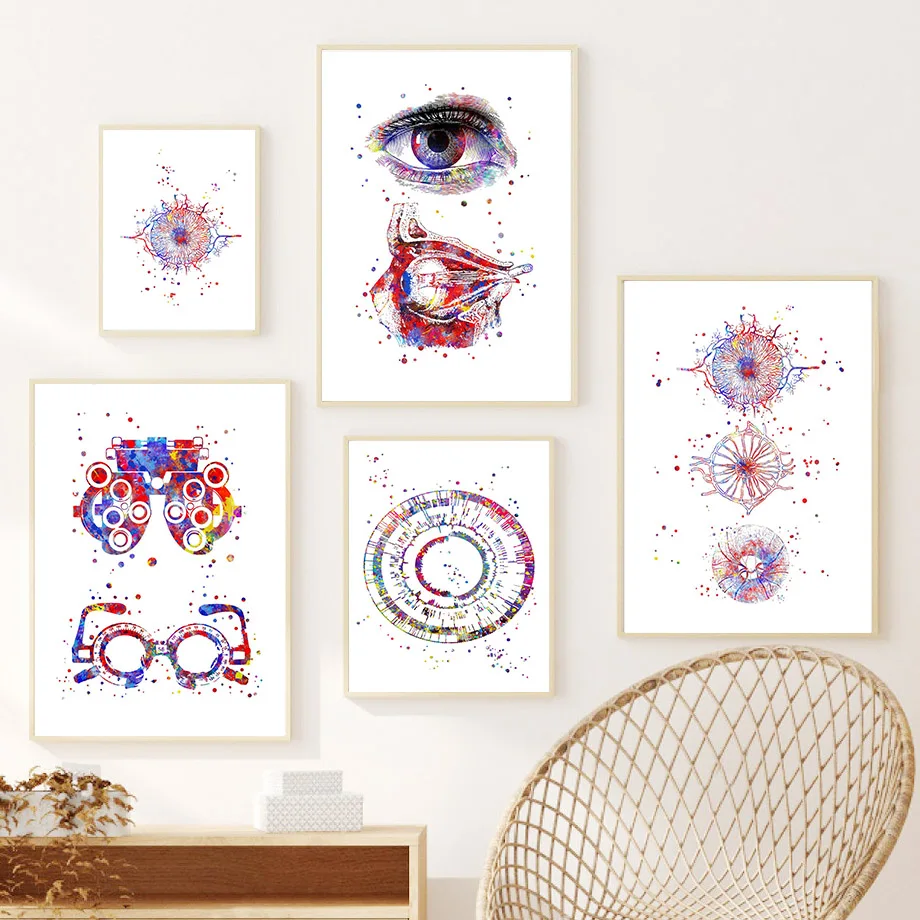A meticulously arranged wall serves as a modern canvas, adorned with five pieces of pastel-hued art on a pristine white background. The centerpiece, prominently situated at the top center, is a detailed drawing of a human eye, featuring the eye's muscle and nerve structure in a side-view slice. Surrounding this focal point are artworks that exhibit intricate spirograph-like designs, predominantly in blue and red tones. To the bottom left is an image featuring a pair of optometrist’s glasses used for lens adjustments, adding a touch of scientific intrigue. Adjacent to this is another piece of optometric apparatus designed for visual focus tests. The artworks vary in size, with three larger pieces and two smaller, square ones, all unified by their detailed, circular patterns. Below the collection, to the left, a wooden accent table peeks into view, while to the right, a rattan clam-style chair adds warmth to the minimalist setting, creating a serene and thoughtfully curated aesthetic.